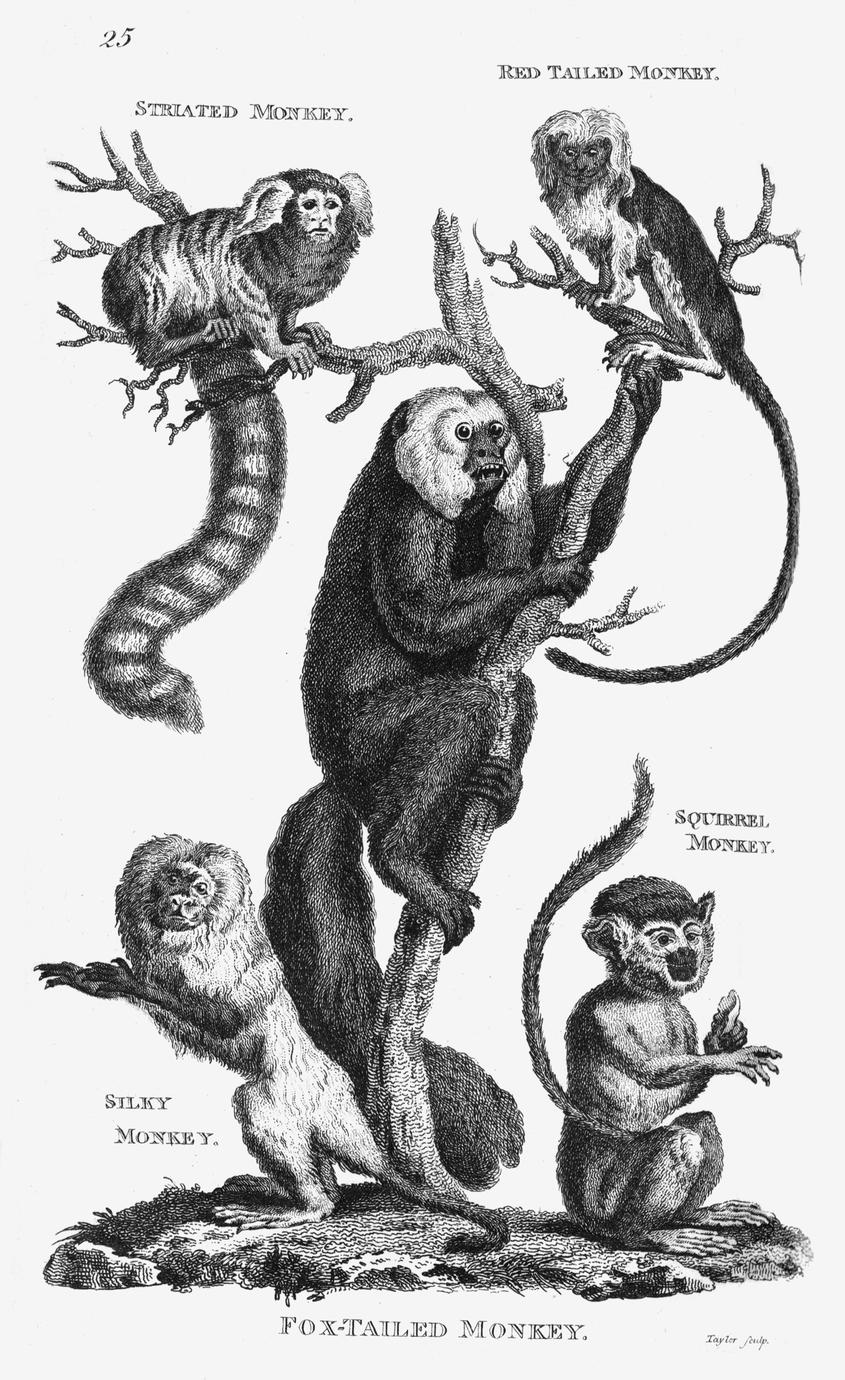The black and white illustration features a detailed sketch of five different types of monkeys, each labeled with their respective names. Central to the illustration is a large tree with various branches supporting the monkeys. At the top left branch, a small striated monkey with a striped fur and bushy tail is perched. Opposite on the top right branch is a red-tailed monkey characterized by its slender tail. Dominating the main trunk of the tree is a larger foxtail monkey, clinging to the trunk with its legs and arms and identifiable by its white face and dark fur. Below, on the bottom left, sits a silky monkey, depicted as smaller and completely white. Finally, to the bottom right, a squirrel monkey is positioned, holding a piece of fruit. The illustration appears to be page 25, indicated by the number at the top of the page, and is set against a white background.